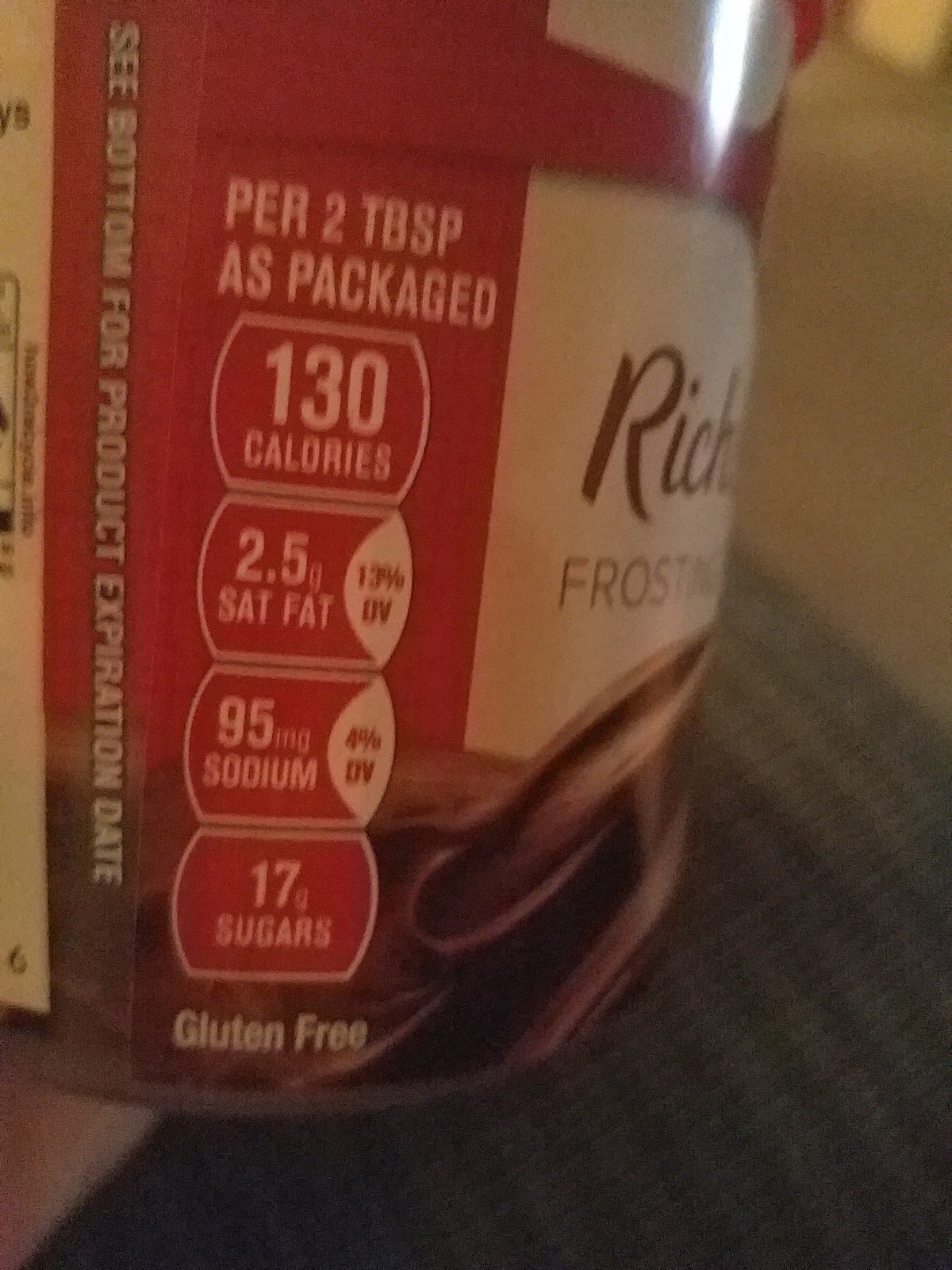This image is a close-up shot of a canister of chocolate cake frosting, held by someone. The label predominantly features a red main body with a tan section on the side, displaying the words "rich" and "frosting" in brown lettering. The label includes nutritional information within four red bubbles with white lettering, where each bubble has flat tops and bottoms with rounded sides. From top to bottom, the bubbles display the following information: 

1. 130 calories ("calories" and "130" in white)
2. 2.5 grams of saturated fat (constituting 13% of the daily value)
3. 95 milligrams of sodium (potentially representing 4% of the daily value)
4. 17 grams of sugars

Above these bubbles, it states "per two tablespoons as packaged." The bottom part of the label confirms the product is gluten-free. Additionally, in a vertical orientation, it instructs to check the bottom of the canister for product expiration dates.